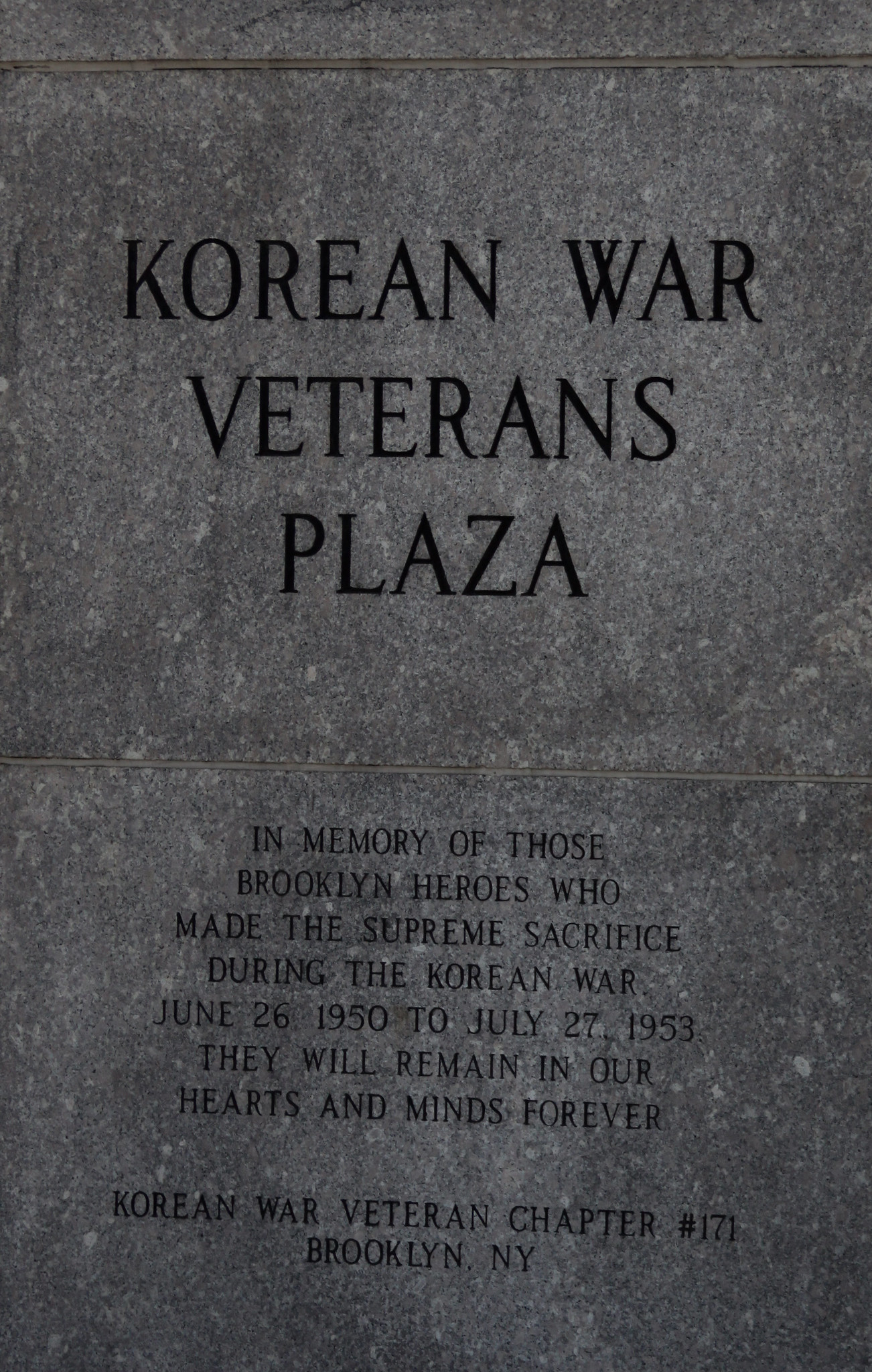The image depicts a memorial plaque embedded in a gray stone monument, honoring Korean War veterans from Brooklyn, New York. The top of the plaque features the black engraved text "Korean War Veterans Plaza." Below this, it bears the inscription: "In memory of those Brooklyn heroes who made the supreme sacrifice during the Korean War, June 26, 1950 to July 27, 1953. They will remain in our hearts and minds forever." At the bottom, the plaque reads "Korean War Veterans Chapter Number 171, Brooklyn, New York." This solemn tribute commemorates the bravery and sacrifice of local heroes during the Korean War.